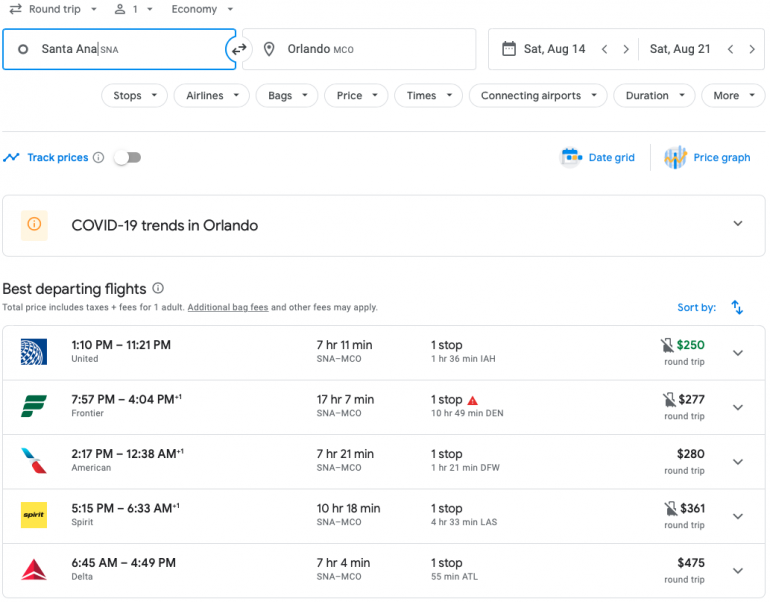The image features a screenshot of a travel booking webpage displayed on a computer screen. At the top of the page, the search criteria specify details for a round trip for one person in economy class, traveling from Santa Ana to Orlando. The travel dates are set from Saturday, August 14th to Saturday, August 21st.

Below the travel search criteria, a row of icons and buttons allows users to filter options by stops, airlines, bags, price, times, connecting airports, duration, and more. Toward the upper part of the screen, there is an option labeled "Track Prices," displayed in blue, though it is turned off. Next to it, "Date Grid" and "Price Graph" are both highlighted in blue, indicating they are active features.

A small circular icon with an "i" inside provides information about COVID-19 trends in Orlando. Beneath this, the webpage displays sections for the best departing flights. The total price, which includes taxes and fees for one adult, is shown, with a note that additional baggage and other fees may apply.

An itinerary summary is visible further down the webpage, providing a detailed breakdown of the selected flights and travel details.